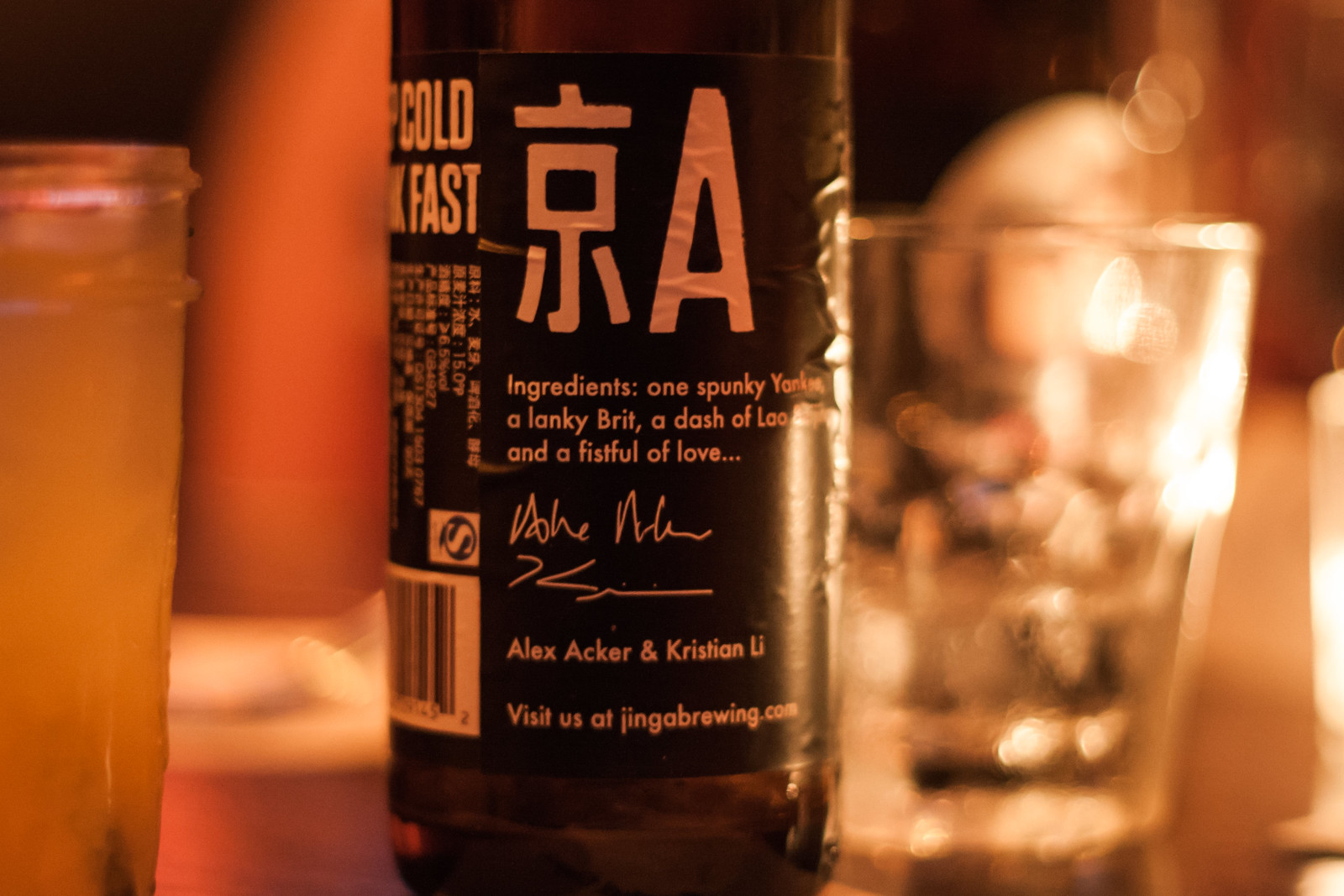The image showcases a rectangular photograph with a warm, orange tint, predominantly focusing on a dark brown bottle situated at the center. The bottle, potentially a beer bottle or a tea bottle, features a black label with white and orange text. The top part of the label displays two undecipherable characters, likely in Japanese or Chinese. Below these, "Ingredients" is written in English, followed by a whimsical list: "One spunky Yankee, a lanky Brit, a dash of loo, and a fistful of love." Below the list are signatures with the names Alex Archer and Christian Yu, and the website "visit us at jinglebrew.com." The left side of the label features the words "cold and fast" along with a barcode and additional text that can't be clearly made out.

Flanking the central bottle are blurred objects: on the right, there's what appears to be a glass containing ice cubes and an unidentified liquid, and on the left, a tall, possibly frosted or condensation-covered glass or candle. The background is predominantly black, adding to the focus on the central bottle and the soft, orange-lit ambiance of the scene.